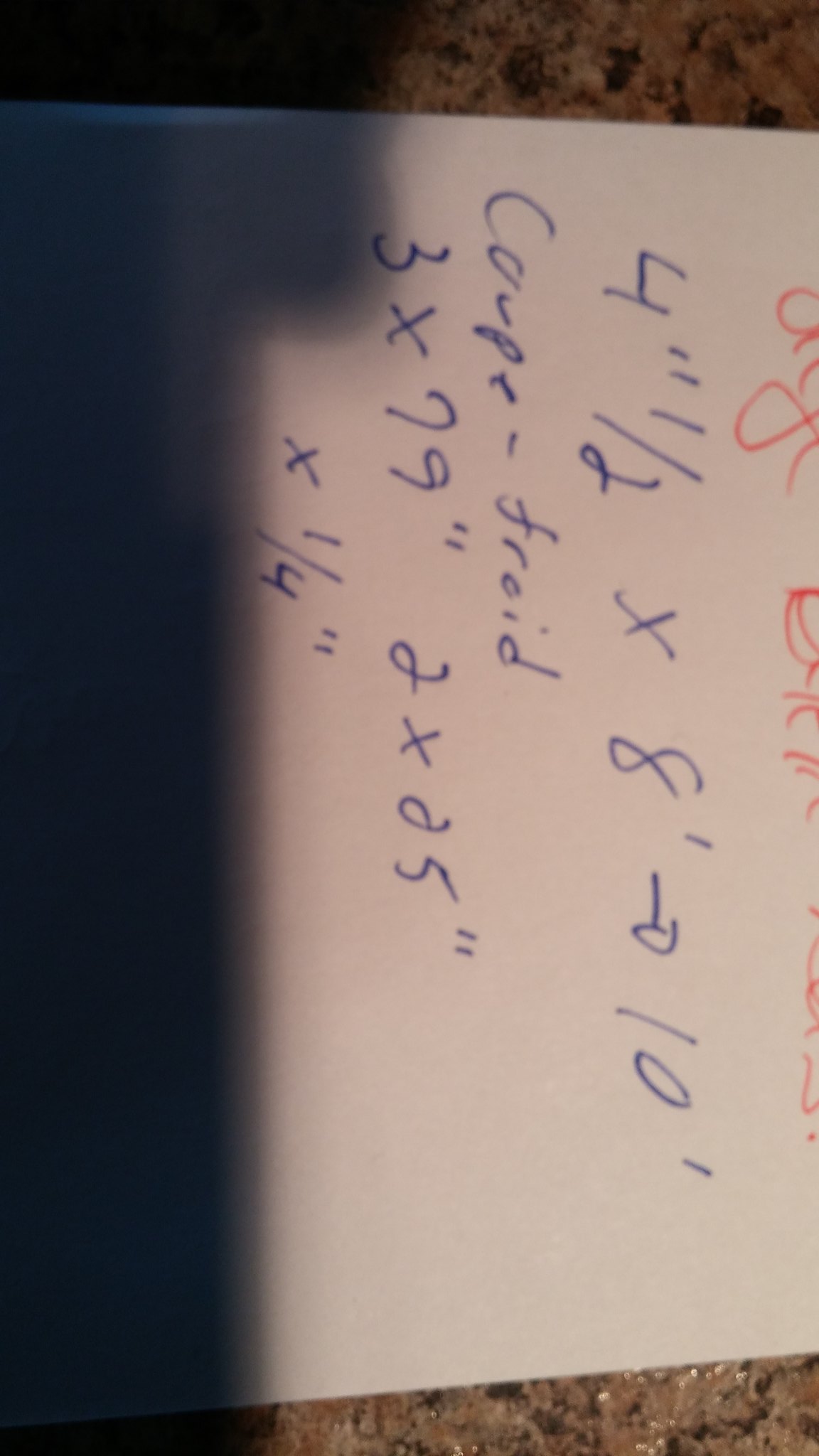The image showcases a small piece of white paper, positioned sideways on a pinkish granite surface with black speckles. The paper measures just a few inches in width and height, clearly not a full-sized sheet. The top portion of the paper is partially cut off but features cursive handwriting in red ink, which is illegible due to the cutoff. Below the cursive writing, written in blue ink, are several mathematical figures: "4 inches 1/2 x 8/arrow to a 10". Further down, there's some text that is difficult to decipher, followed by additional numerical expressions: "3 x 79, 2 x 25 x 1/4". The photograph appears to have been taken from an angle that provides a clear view of both the markings on the paper and the distinctive granite background.